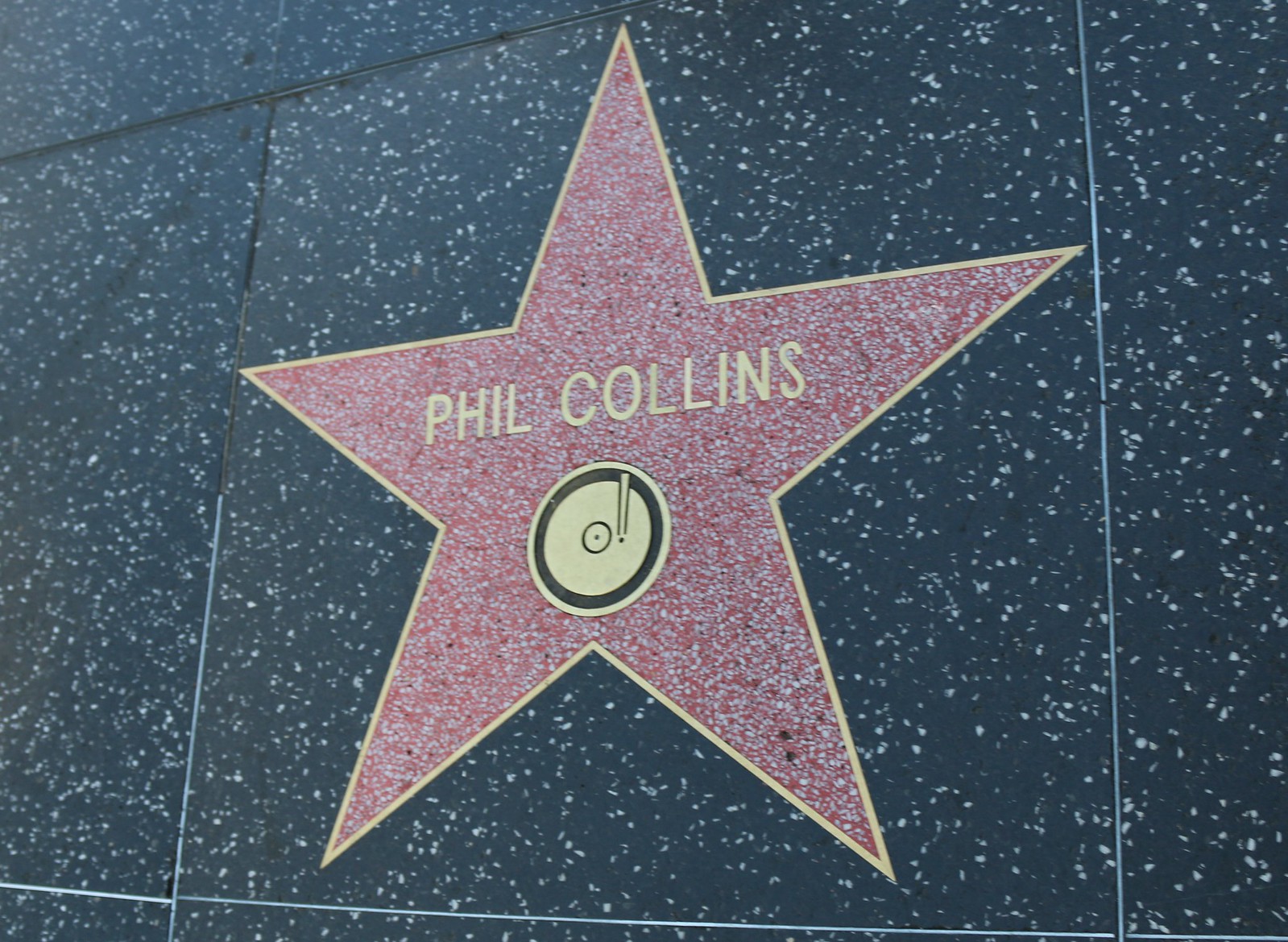This image showcases Phil Collins' star on the Hollywood Walk of Fame, prominently occupying its square on the iconic walkway. The floor is a striking black granite adorned with white speckles, creating a shimmering effect. Phil's star itself features a deep red interior accentuated by a gold outline, and his name is prominently displayed in bold letters. Beneath his name is a symbolic representation of a yellow record with black trim, denoting his achievements in the recording industry. Surrounding Phil Collins' star are other black granite squares, though no other stars are visible in this close-up shot. The intricate details include white grout lines highlighting the star’s placement and the sharp, well-defined points of the star corners. The overall scene captures the prestige and recognition associated with the Hollywood Walk of Fame, honoring Phil Collins' legacy as a celebrated recording artist.